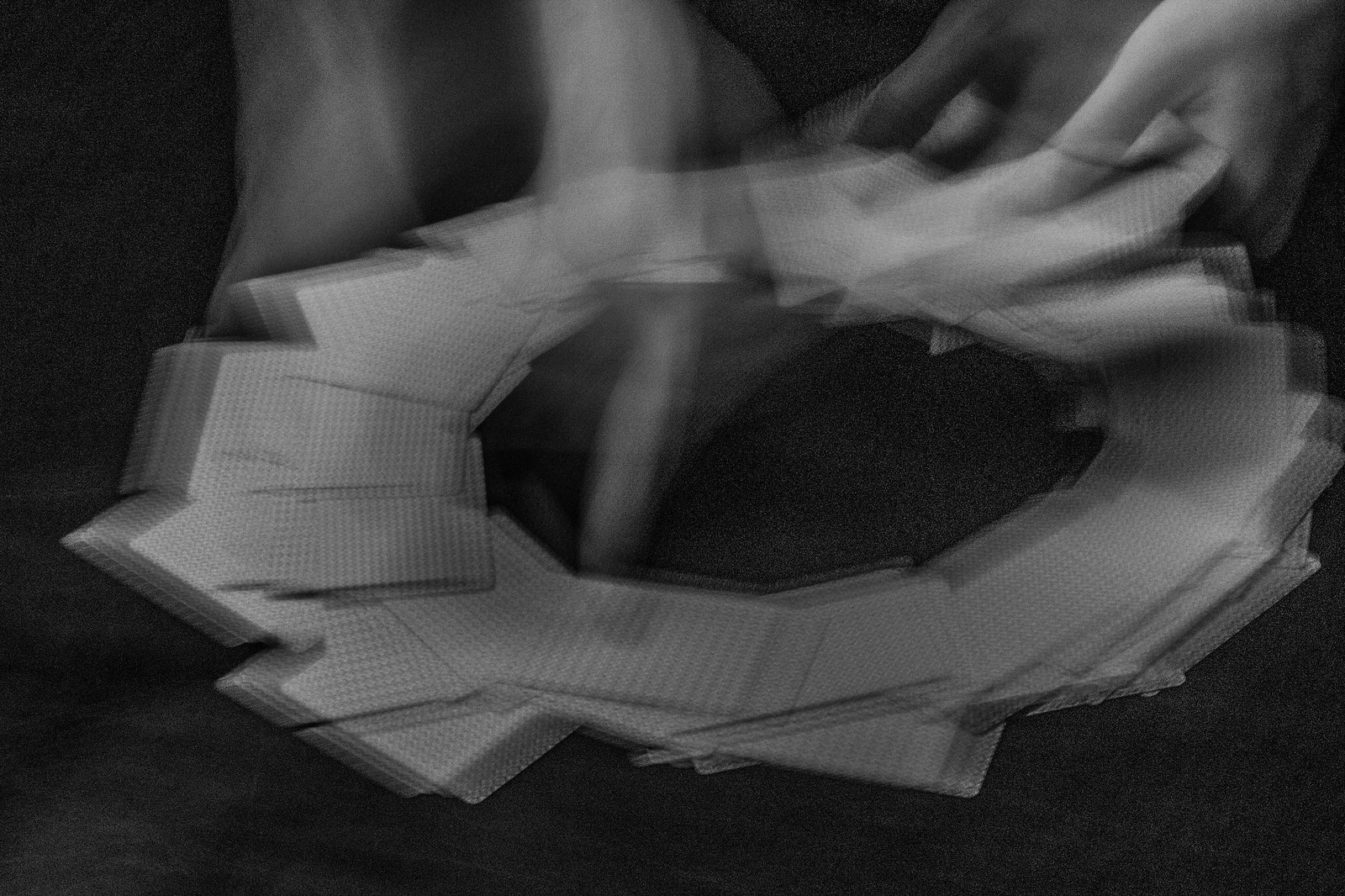In this black-and-white image, a series of white playing cards are arranged in a circular pattern. The cards, adorned with intricate designs, form a striking visual against the dark background. A hand, captured in a state of motion blur, interacts with the circle of cards. The hand is most discernible towards the right corner of the image, while its rapid movement elsewhere creates ethereal streaks of light, giving the scene a dynamic and almost ghostly effect. The overall composition emphasizes the contrast between the stark white of the cards and the deep black of the surface, highlighting the fluid motion of the hand.